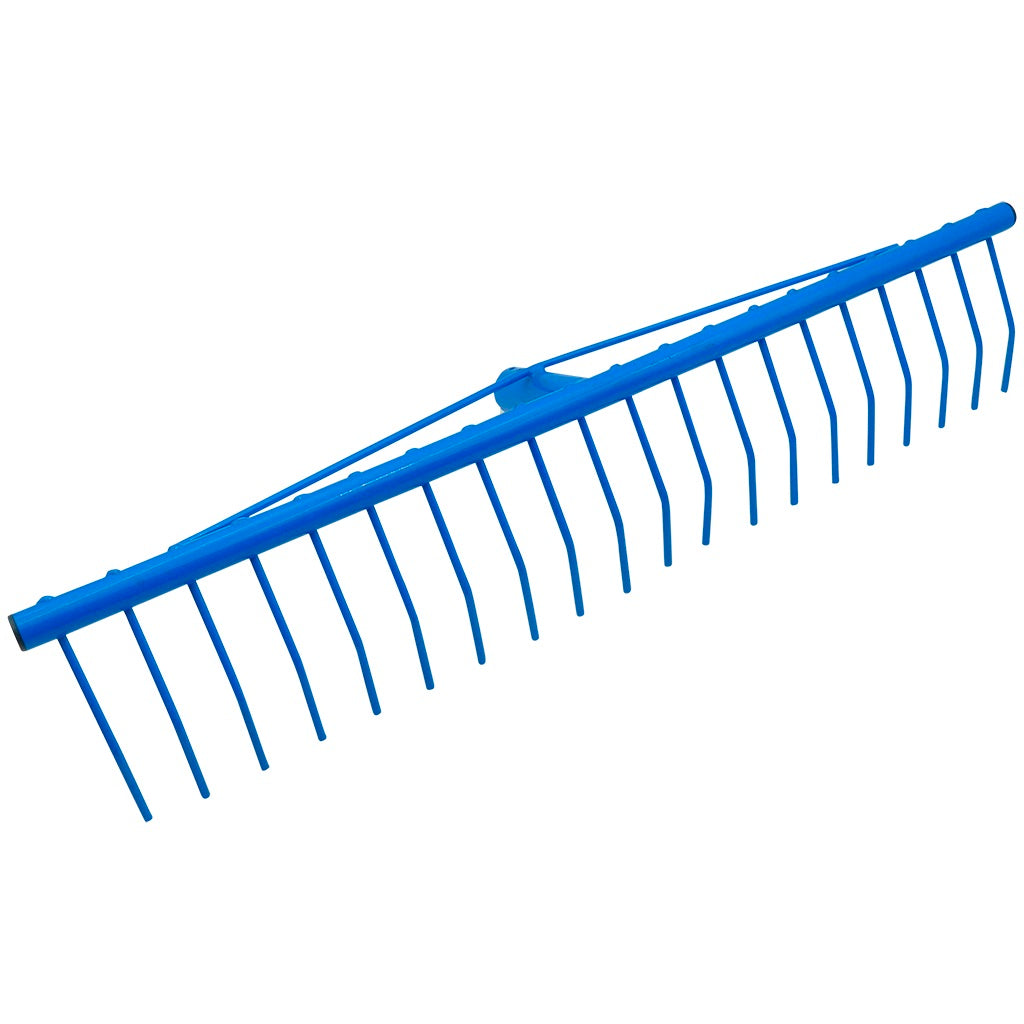The image features a blue rake head against a white background. The rake head has a long, cylindrical blue bar with black end caps and lacks a handle. It is arranged diagonally from the bottom left to the top right of the image. The rake head consists of 20 equally spaced prongs. These prongs, which appear to be bent at approximately a 25-degree angle, extend downward from the main bar and are designed to drag along the ground. At each end of the cylindrical bar are smaller metal tubes that would typically connect to a handle.